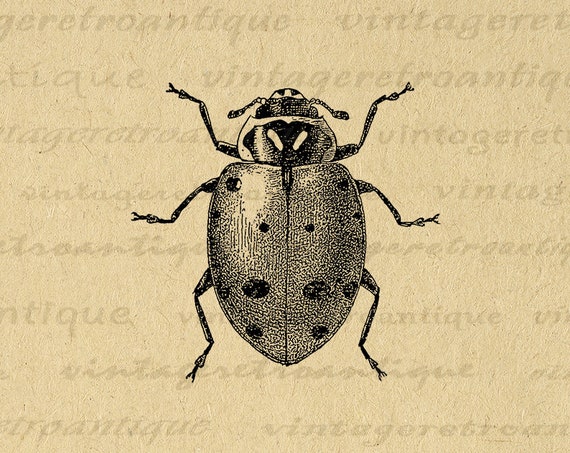This illustration features a detailed pen and ink drawing of a ladybug, presented in a high-contrast black and white style reminiscent of scientific textbook illustrations. The ladybug, identifiable by its distinct, cylindrical body and characteristic black spots, is rendered with simplicity and precision, omitting color to focus on form and details. The background is a creamy, off-white paper texture resembling vellum, enhancing the illustration's vintage aesthetic. This background is overlaid with the phrase "vintage retro antique" repeated across the image in approximately 50 different fonts. This text spans the image like a watermark, giving it a retro feel and possibly serving as a branding element to prevent unauthorized use.